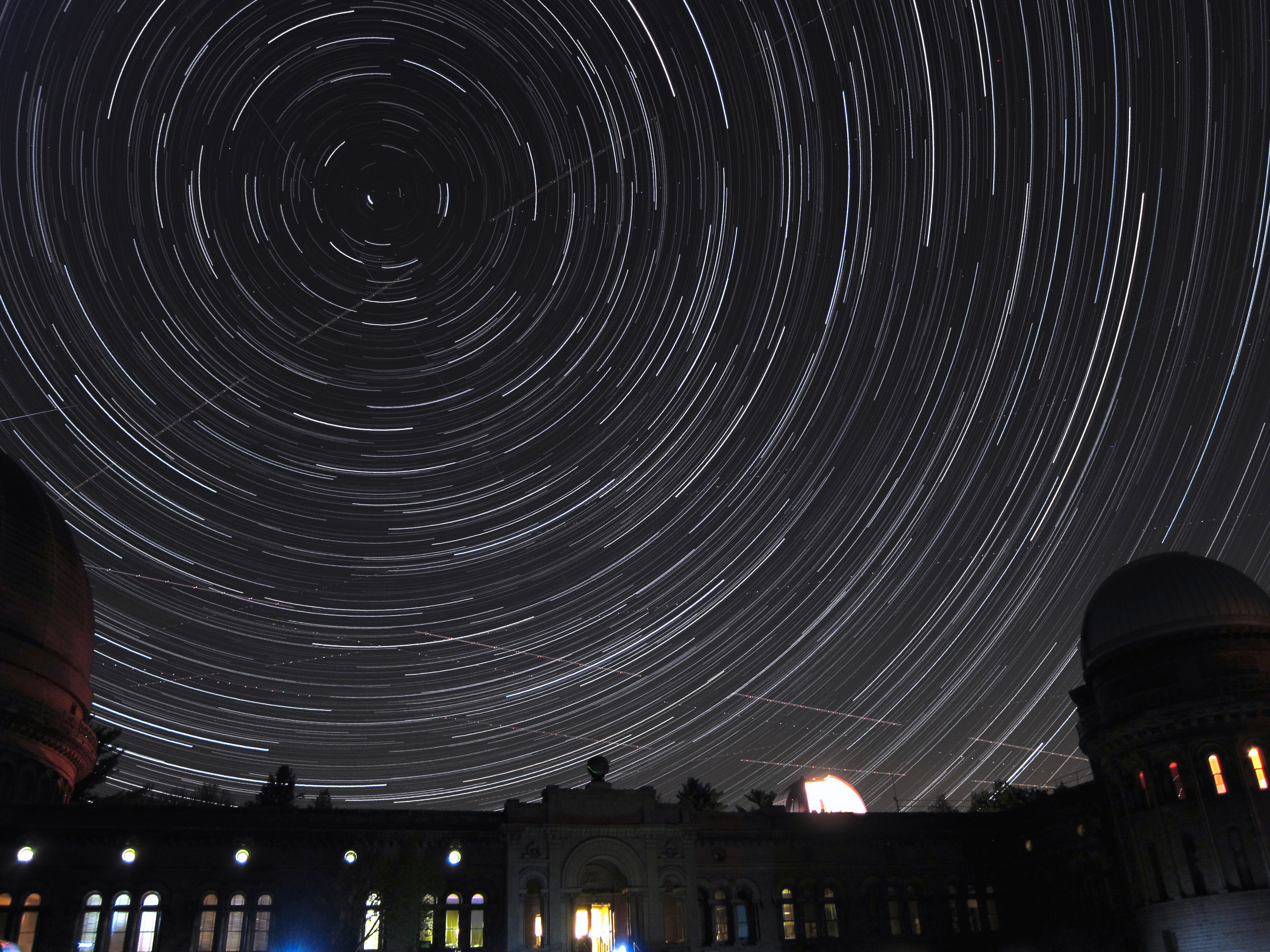The image is a detailed portrayal of a nighttime sky captured through a timelapse or long exposure technique, showcasing the mesmerizing effect of circled, radiating star trails that create a vortex-like appearance above. The sky is predominantly dark with hues of gray and white, interspersed with streaks suggesting the paths of shooting stars. Below this celestial display, there is an elaborate, grand structure resembling an observatory or possibly a museum, constructed from gray stone or marble. The building features multiple domes—one prominent dome on the right and another on the left, the latter with a distinctive reddish-brown tint. The building is dotted with arched windows, emitting a warm glow from within, enhancing the serene yet majestic ambiance of the scene. The overall palette of the image is a blend of somber grays, blacks, and whites, accented by subtle tones of blue, gold, and yellow.